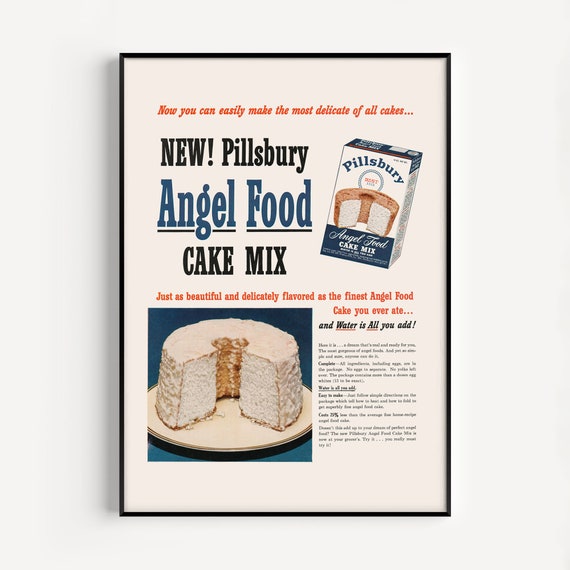The ad is a vertically rectangular print piece with an off-white background and a black frame, casting a slight shadow on the left side. The main feature is an advertisement for Pillsbury Angel Food Cake Mix. At the top, red text declares, “Now you can easily make the most delicious of all cakes,” followed by "new Pillsbury" in black, and "Angel Food" in blue, with "Cake Mix" in black beneath it. To the right of this header, there's an image of the Cake Mix box. Across the center in red, the ad states, “Just as beautiful and delicately flavored as the finest angel food cake you ever ate,” emphasizing simplicity by adding, “And water is all you need,” in black. In the lower left-hand corner, there’s a photograph of a white angel food cake with a slice cut out, showcasing both the exterior and interior of the cake.